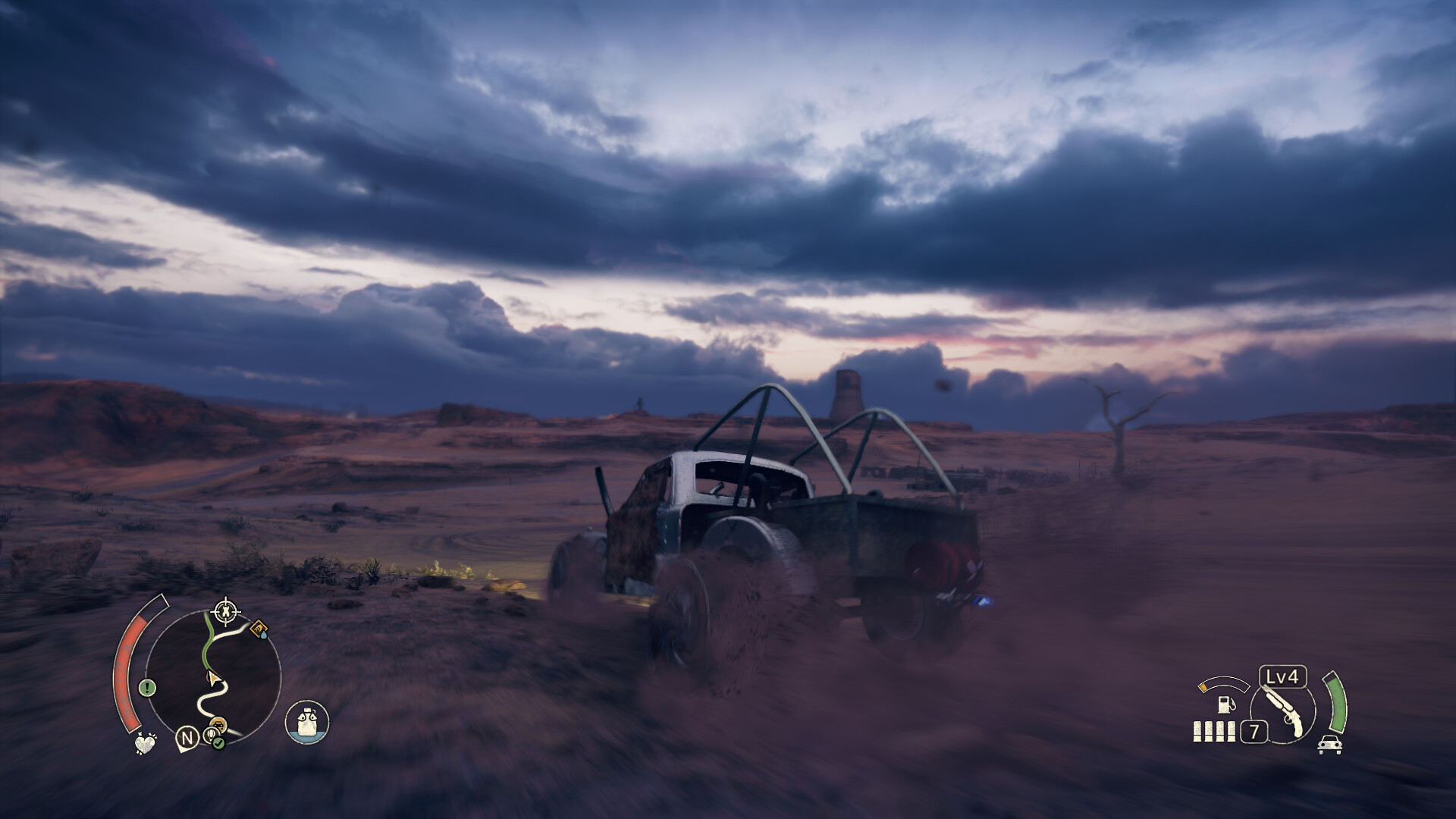In this detailed image from a computer or console racing game, we see a car speeding through a vast desert landscape. The player controls the car, which appears to be navigating the sandy terrain. The game interface displays various indicators: in the lower left-hand corner, a trail with a red bar could signify speed, fuel, or health levels. The lower right-hand corner shows the player is on level four, with nearly depleted gas. Additionally, there is a number seven accompanied by what seem to be bullet icons, suggesting ammunition or power-ups. Also visible is an icon of a car with a green stripe, potentially indicating the car's current speed or status. The overall scene captures the intensity and focus required for desert racing in the game.